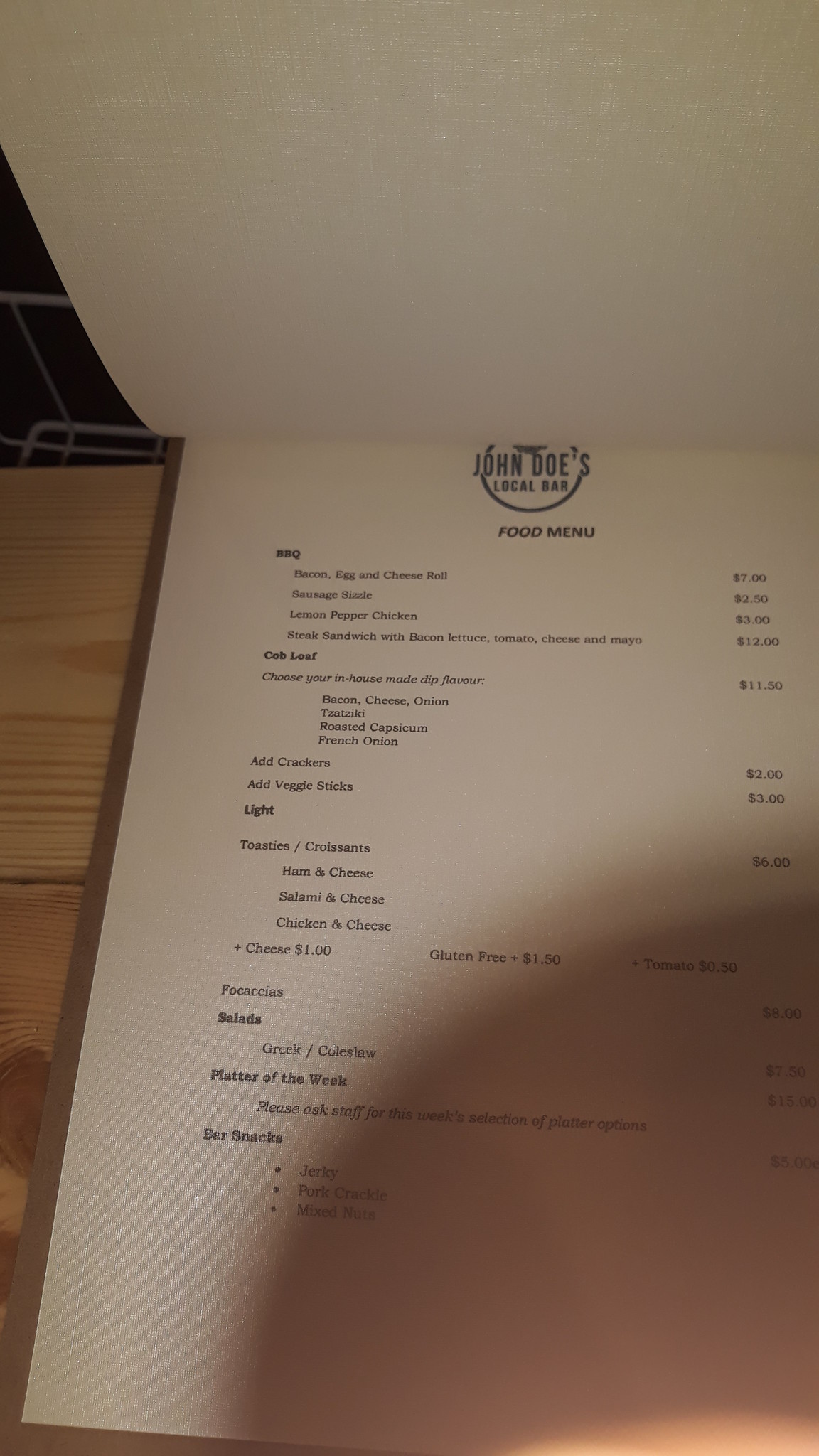This image captures a detailed view of a menu from John Doe's Local Bar, set against a table with a backdrop of black tiles featuring white grout lines. The top page of the menu is held up by a clipboard, allowing a clear view of the layout beneath. At the top of the menu, the establishment's emblem stands out: a circular design with "John Doe's" in large capital letters, where the "J" and "S" extend beyond the circle's rim, accompanied by "LOCAL BAR" in smaller capital letters within the circle. The menu is organized into various sections, each with prices listed to the right. The sections include "Barbecue," "Cob Loaf," "Light," "Salads," "Platter of the Week," and "Bar Snacks." A shadow cast by the photographer is noticeable over the bottom right corner of the menu, adding a touch of realism to the scene.